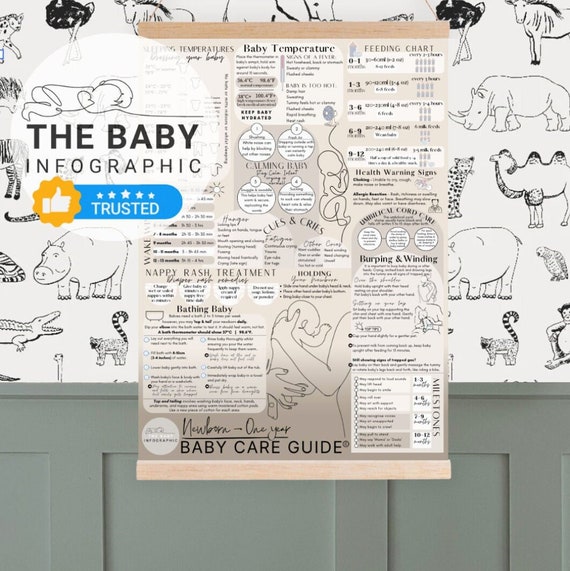This image depicts a baby care guide poster displayed on an animal-themed wall, which is divided into a black and white wallpaper of zoo animals like rhinos, camels, alligators, ostriches, and monkeys on the top, and grey painted wooden paneling below. The poster, framed by flat wooden edges at the top and bottom, is an infographic packed with detailed information on infant care, including feeding charts, baby temperature guidelines, rash treatment instructions, and tips on bathing, burping, and feeding a baby. In the top left corner of the infographic is a black and white line drawing of a baby lying down, with the text "The Baby Infographic" next to it. Adjacent is a golden badge featuring a thumbs-up symbol and five stars with the word "Trusted" in white text within a blue, pill-shaped background. The scene appears to be set in a doctor's office or nursery, suggesting a trusted and informative environment for baby care.